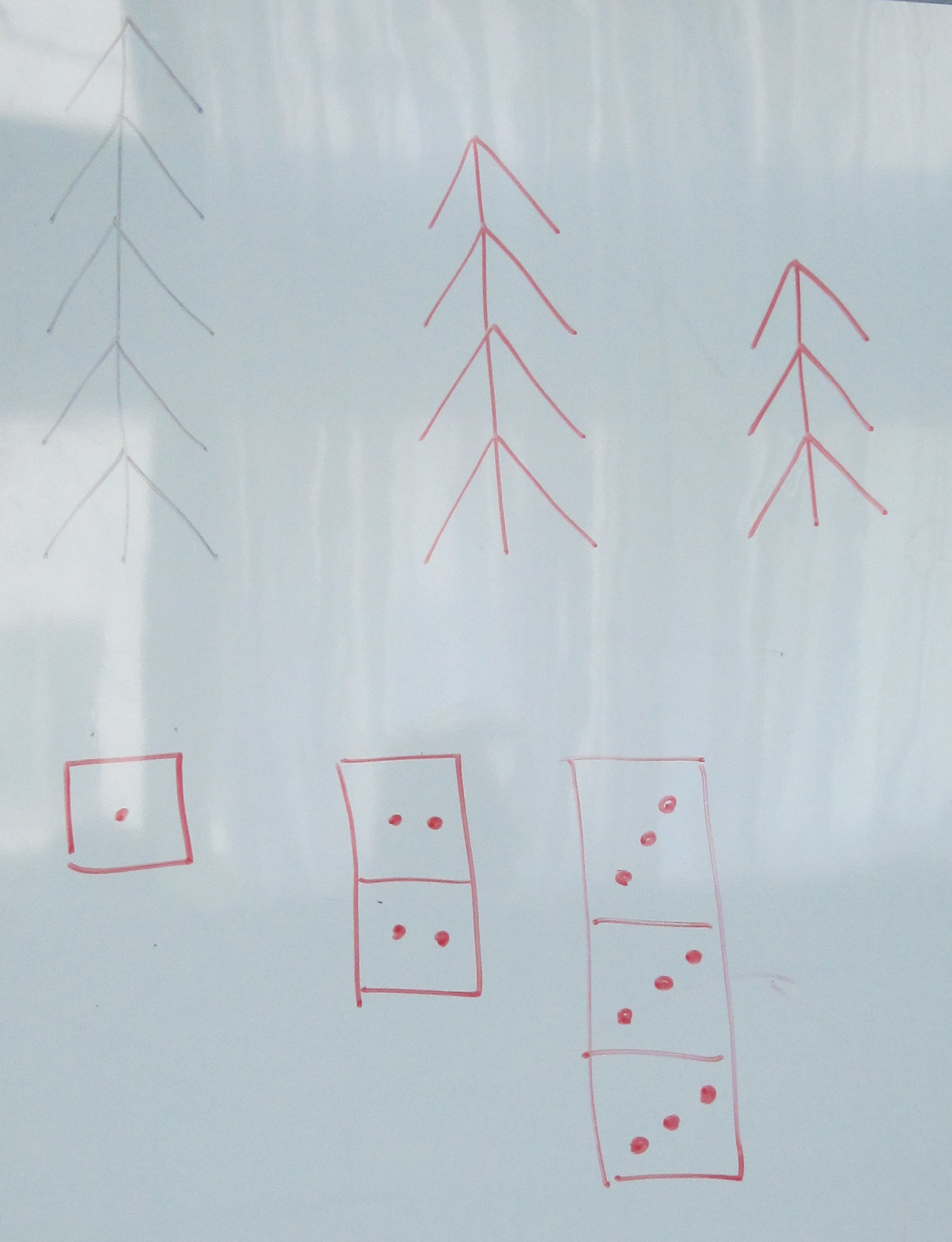This photograph captures a piece of white paper adorned with whimsical red marker doodles, likely created by a child. The upper portion of the paper features a trio of rudimentary stick-figure trees. Each tree is depicted with a vertical line as the trunk, topped with a series of inverted V shapes resembling the peaks of triangles. These trees vary in height, with the tallest on the left and progressively shorter ones to the right.

Beneath the trees, a series of domino-like drawings can be seen. Directly under the tallest tree is a single square with a dot at its center. To the right of this is a pair of adjacent squares, each containing two central dots. The final set, under the shortest tree, consists of three connected squares, each with three diagonal dots ascending upwards.

The paper itself appears to have a somewhat transparent quality, suggesting it may be held against a light source or suspended, allowing subtle shadows to be visible through it. This detail adds an extra layer of depth and texture to the simple, yet charming artwork.